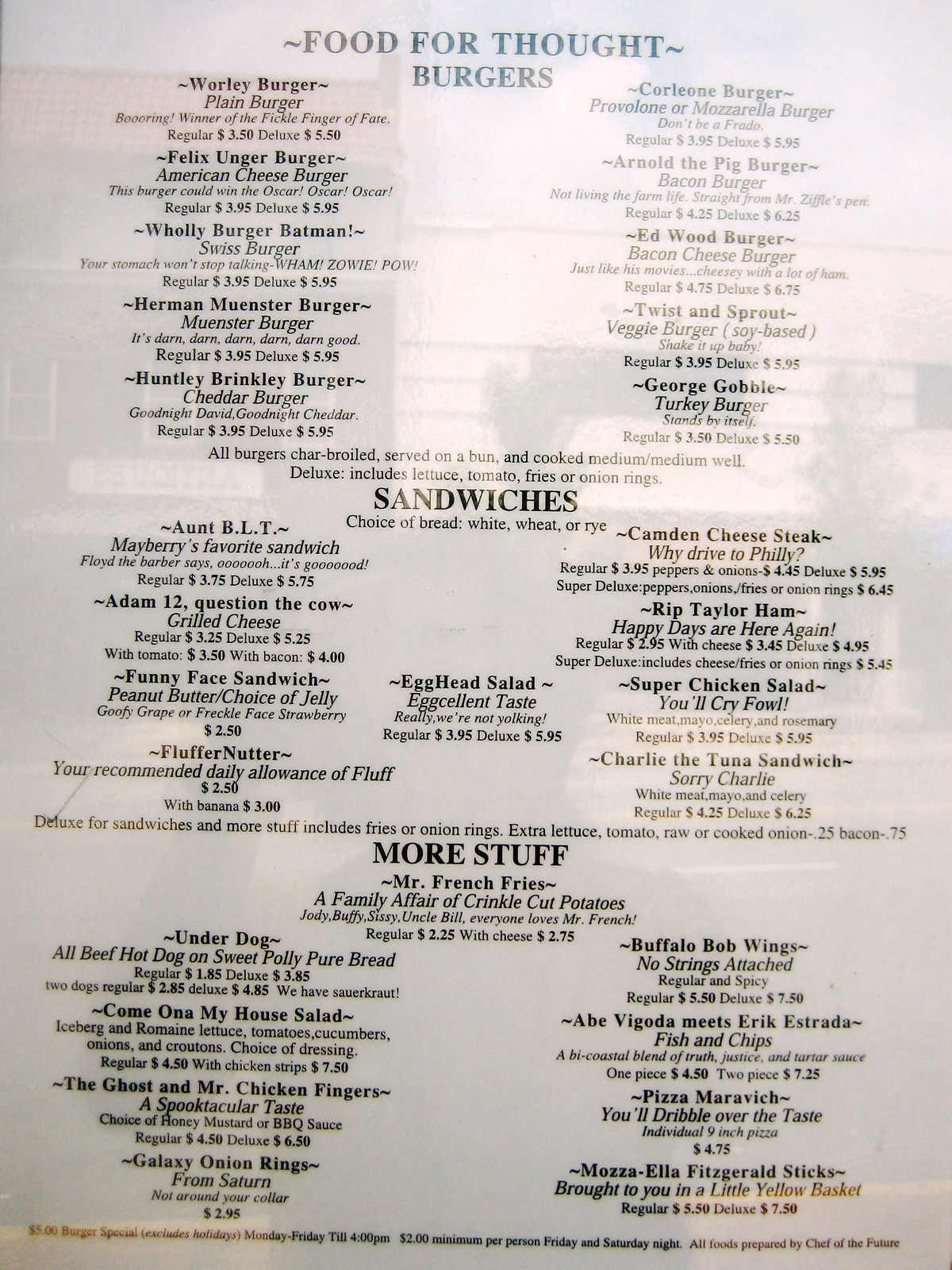The photograph captures a reflective view of a menu taken from inside a window. The reflections reveal surrounding buildings, trees, and the person taking the photograph, creating a layered and introspective composition.

At the top of the menu, the title "Food for Thought Burgers" is prominently displayed in dark blue text. Below this, the burgers are listed in black text, arranged neatly in two centrally-aligned columns. Each burger description is centered for clarity.

Following the burger section, a note in black text clarifies: "All burgers are charbroiled, served on a bun, and cooked medium to medium well. Deluxe includes lettuce, tomato, fries, or onion rings."

Further down, the menu transitions to a section titled "Sandwiches" in large black text. Below this title, it specifies: "Choice of bread: white, wheat, or rye." The sandwiches are listed in three columns, with the left and right-most columns featuring centered text. Remarkably, the middle column contains a single item: the "Egghead Salad Sandwich."

At the bottom of the menu, another section in large font introduces more items. Underneath, in centered text, the phrase "Mr. French Fries - A family affair of crinkle cut potatoes" is written. The section concludes with two columns of additional menu items, again presented in centered text.

The well-organized structure and detailed descriptions are designed to capture the reader’s attention and provide clear, easy-to-read options.